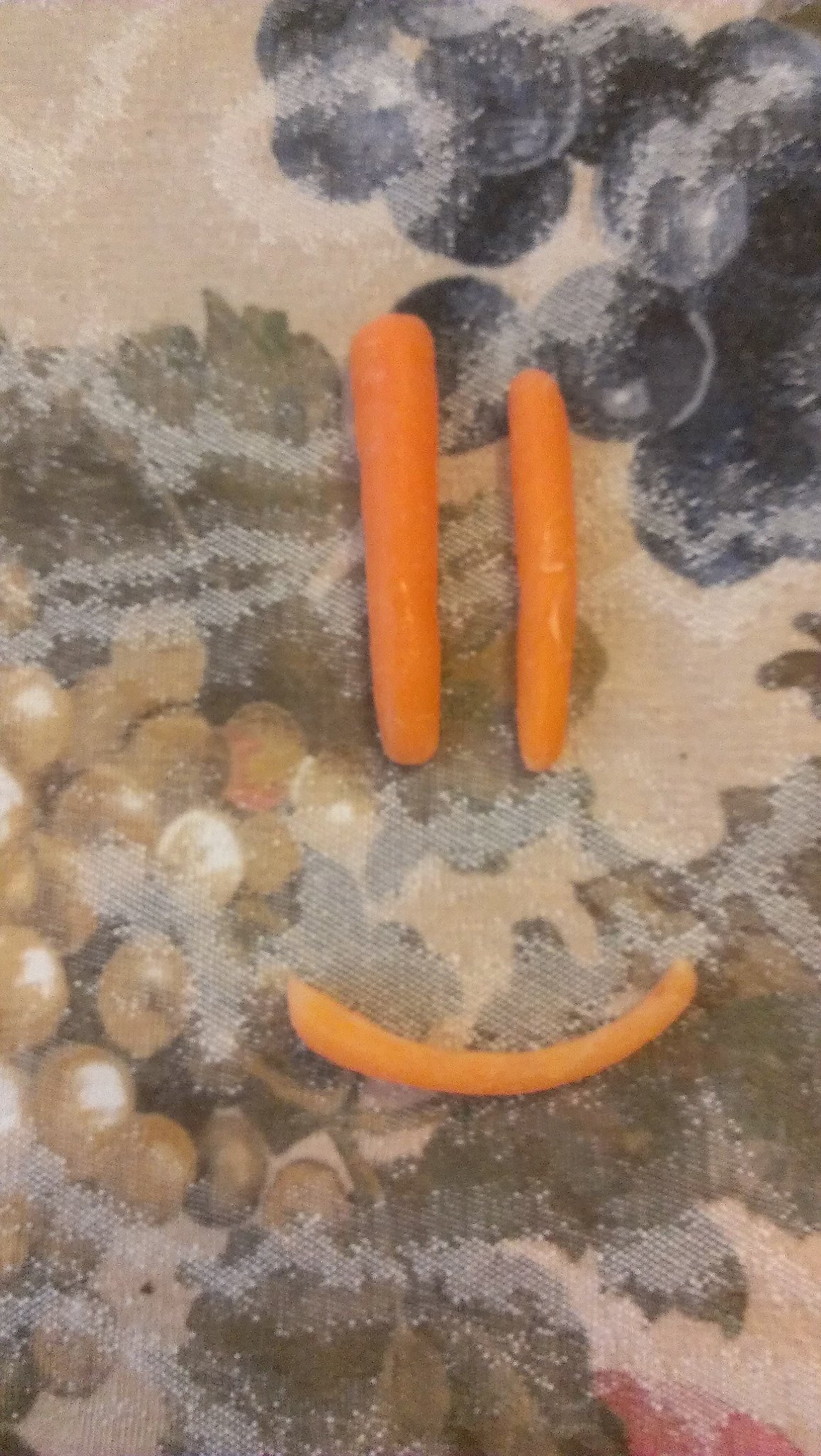This overhead image captures a playful arrangement of orange carrots forming a smiley face on a muted, tan tablecloth adorned with a grape motif. The eyes are represented by two vertical baby carrots, with the right eye being noticeably smaller than the left. Positioned below is a curved piece of shredded carrot forming the mouth. The detailed tablecloth features patterns of green grape clusters surrounded by grape leaves, with larger purple grapes visible in the upper and lower right corners. The composition effectively juxtaposes the vibrant orange carrots against the intricate, softly colored grape-themed backdrop, creating a cheerful and visually engaging scene.